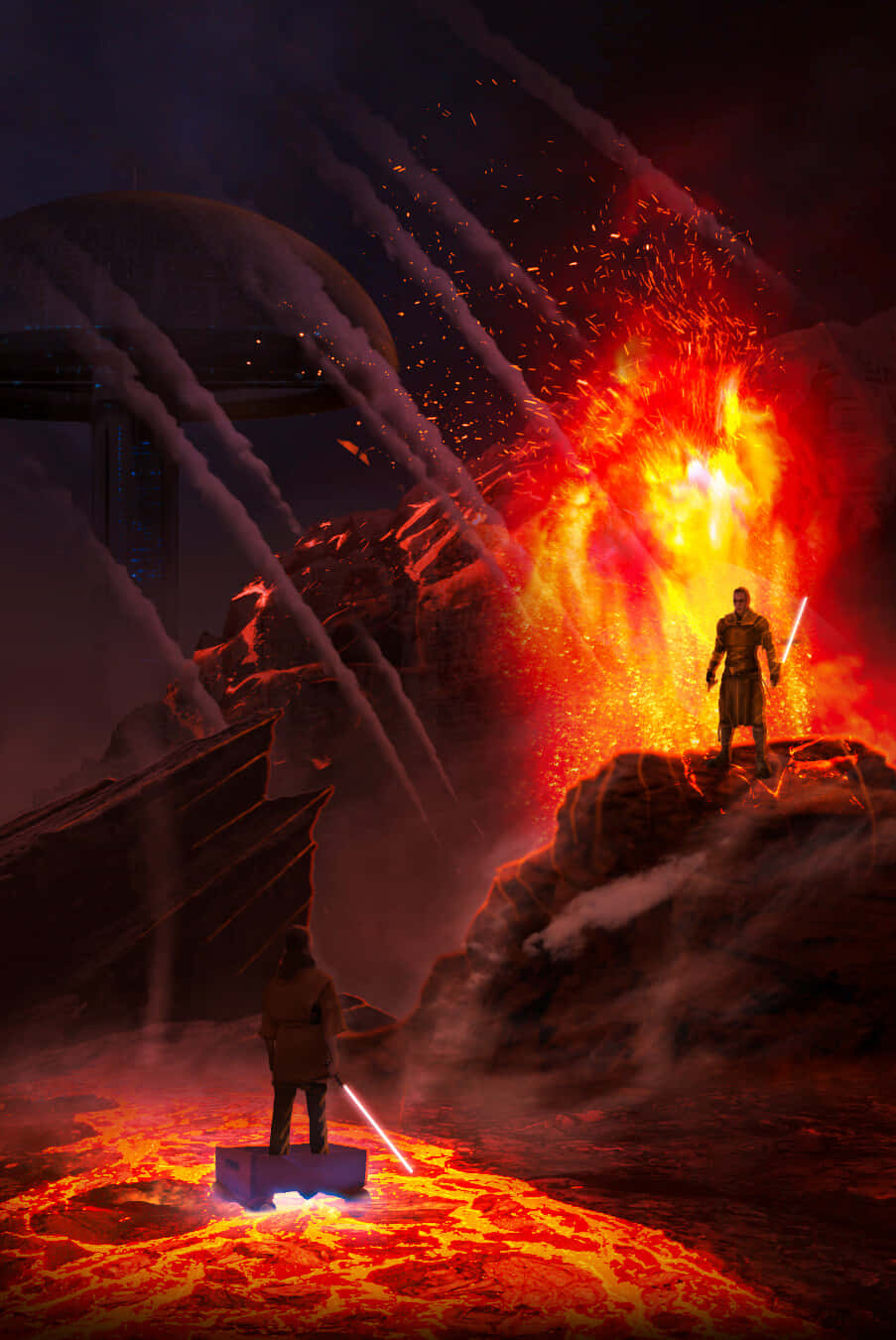The computer-generated image, potentially from a video game inspired by the Star Wars genre, depicts a dramatic confrontation against a dark, fiery background. On the right side of the image, a menacing volcano appears to be spewing bright orange and yellow lava, casting an ominous glow. Trails of gray smoke rise from the eruption, adding to the chaos. In the foreground, a person clad in a brown jacket stands on a rectangular block amidst the lava, wielding a white lightsaber. This figure is positioned centrally, with their back facing the viewer. To the right, on a rugged mountain or cliff, another figure is visible, also holding a white lightsaber and dressed in similar brown attire. On the left side of the background, a distinctive mushroom-like building tower can be seen. The overall scene is dark, emphasizing the fiery explosion and the intense standoff between the two characters, readying for a duel.